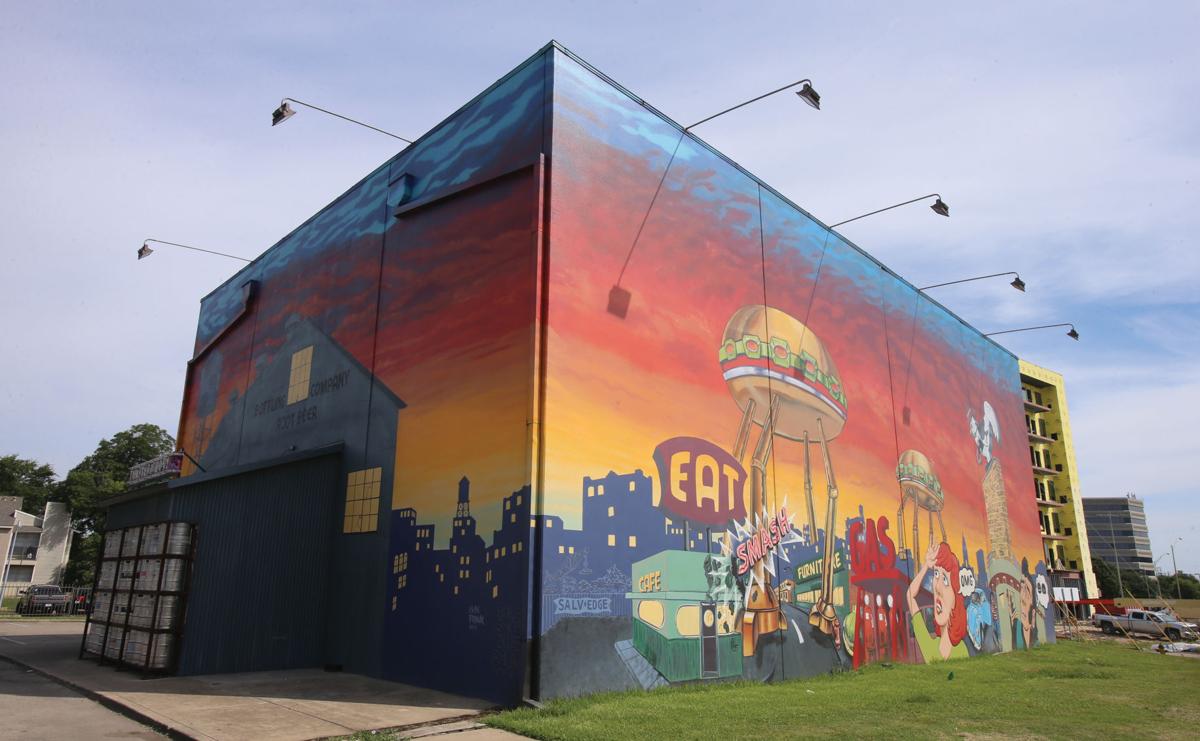This photograph captures the corner of a large two or three-story rectangular building, illuminated by hanging lights attached to poles extending from the roof. The building's distinctive feature is a vibrant mural that spans both visible facades, designed to resemble a comic strip. The mural showcases a surreal cityscape beneath a gradient sky of pink, orange, and burnt red. Prominent in the scene are colossal cheeseburgers with robot legs, invading the city. Panicked residents, painted in a 1950s style, gaze upward in astonishment. The mural also features a restaurant with the text "Eat" prominently displayed, hinting that the building might be a themed establishment, possibly a restaurant. The mural's fantastical elements, colorful palette, and detailed urban setting make it an eye-catching piece of street art. The immediate surroundings include grass on the right side and a concrete area with an entrance on the left, suggesting a well-trodden path for visitors.